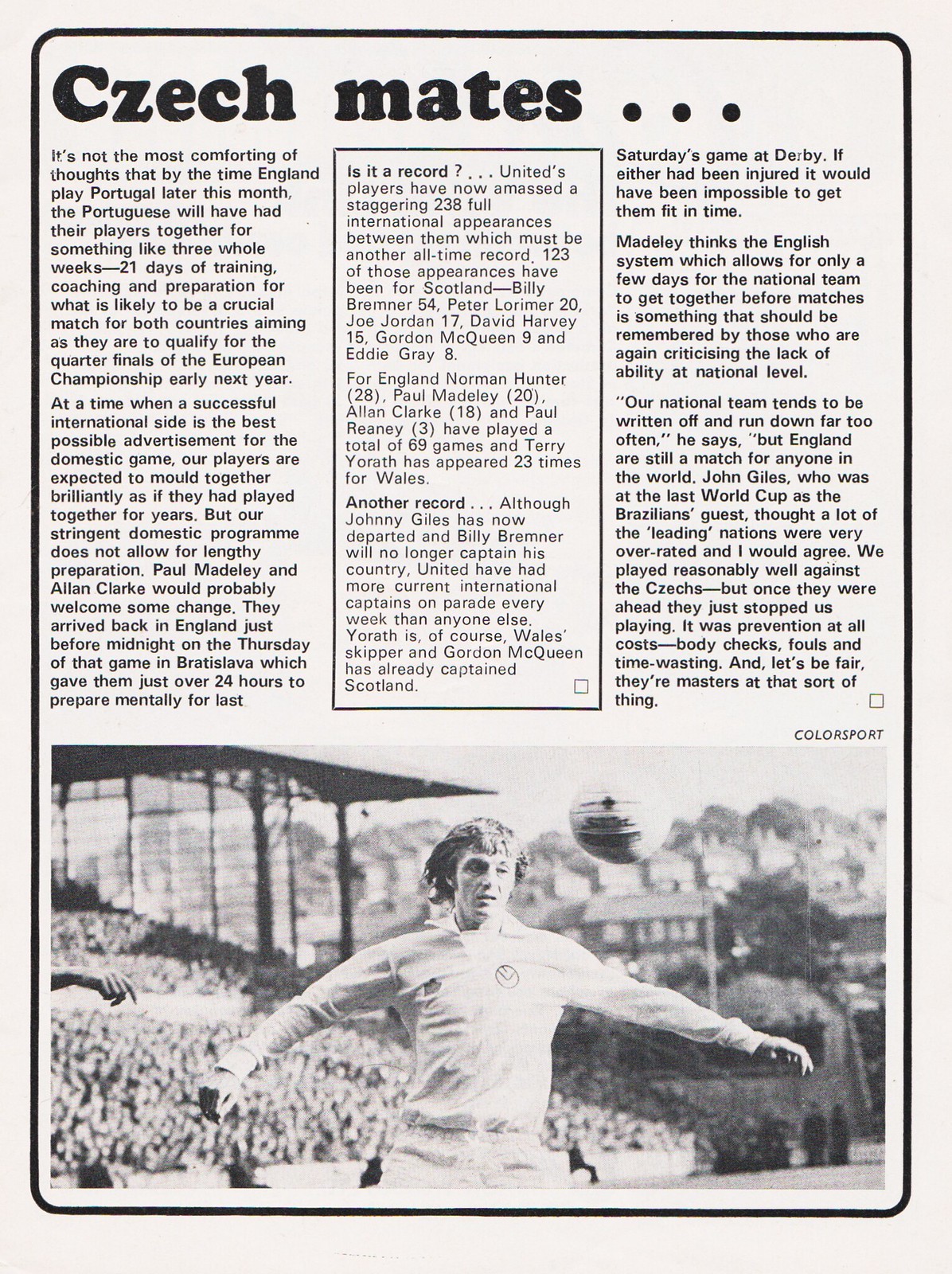The image showcases a segment from a newspaper sports page, aptly titled "Czech Mates." The article, printed in fine black text on a plain white background, details a surprising victory by the Czech team in a soccer match. The article is organized into three columns. At the bottom, a black-and-white photograph captures the defining moment of the game. In the photo, an older soccer player with longish hair is depicted with outstretched arms, catching a soccer ball on his chest. His right arm is mostly straight but angled slightly downward, while his left arm is curved inward and down. A large crowd watches intently from the background. The article also mentions the significance of upcoming matches for England and Portugal, noting the extensive preparation time that the Portuguese team has had, which adds a layer of intensity to the narrative.